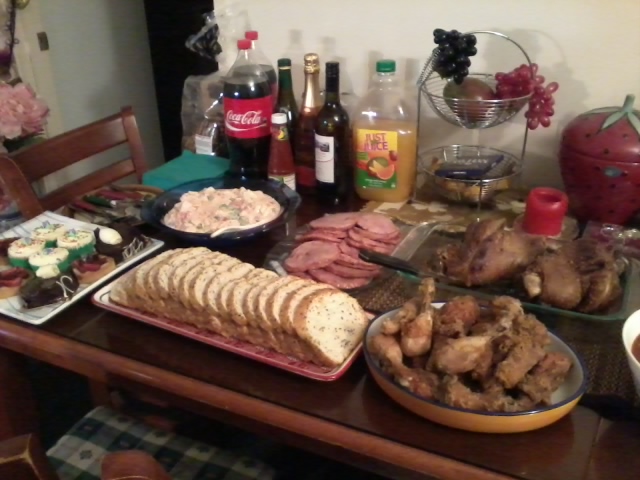The image depicts a richly laden square wooden table in a room with white walls and a black door in the top left background. A dark brown wooden chair is tucked into the left side of the table. Behind the chair, pink flowers are visible against the white wall, and in the foreground on the floor is a green and white checkered mat.

The table is densely covered with various foods and drinks. At the back end are two Coca-Cola bottles, three wine bottles, and a juice bottle. A fruit basket containing what seems to be artificial blackberries, grapes, and a mango is positioned next to these. A distinct strawberry-shaped container with black dots is on the right side of the table.

In the center, there is a tray of sliced meats that appear to be salami, flanked by other bowls - to the left, a black bowl presumably holding porridge or potato salad, and to the right, cooked meat slices. In the bottom right corner is a large plate stacked with fried chicken legs and wings. To its left, a sliced loaf of bread leans slightly to the side. The bottom left corner features either blurry sushi rolls or cupcakes. 

Additional details include green napkins and utensils placed near the brown chair and a dessert plate with cupcakes and brownies situated around the middle left section of the table. The random placement of items suggests a casual, indoor dining setting, perhaps a kitchen or dining room prepared for a substantial meal. The color palette includes tan, light pink, brown, purple, orange, red, and white, complementing the vibrant assortment of food and drink.